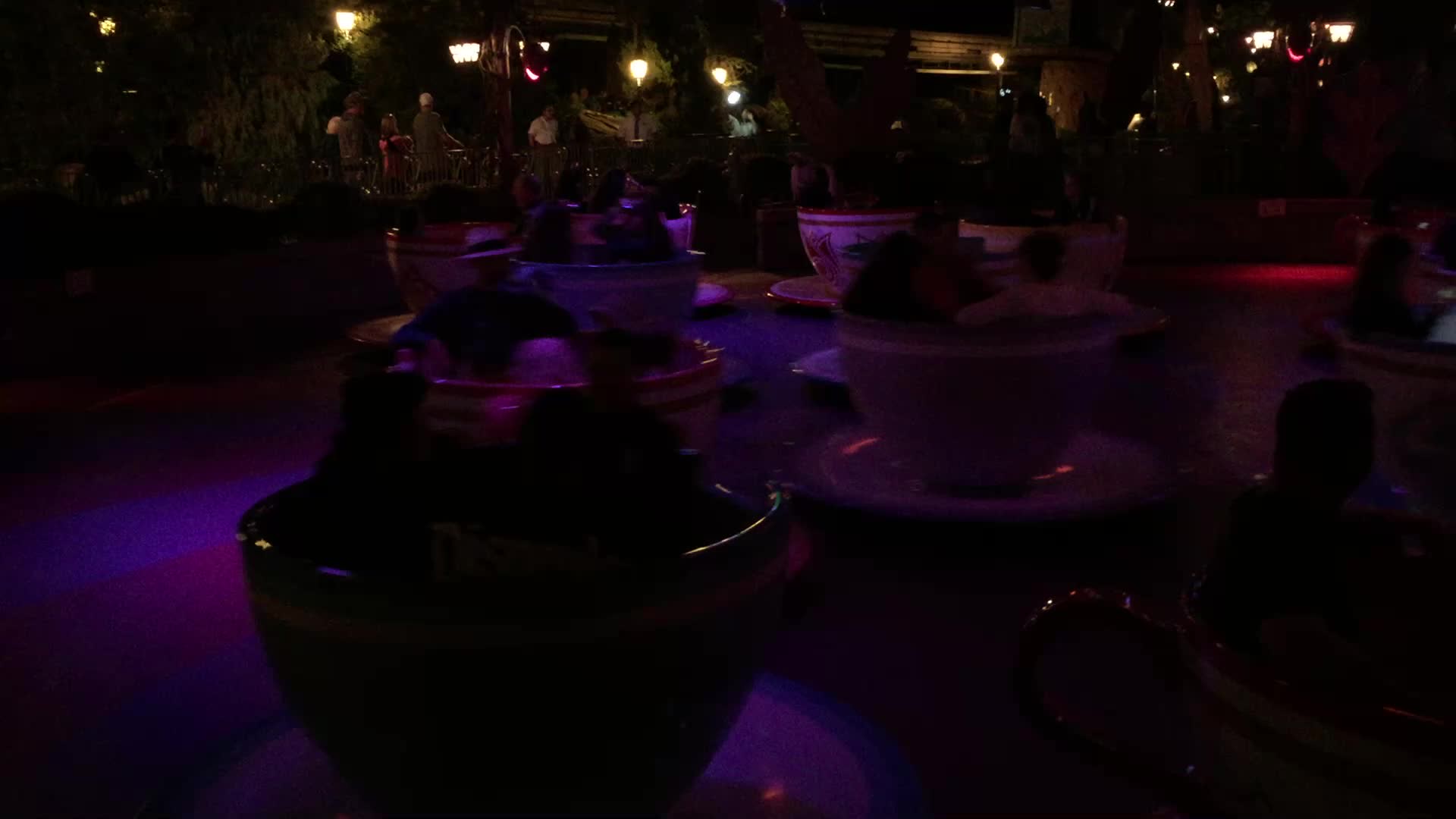In this very dark photograph, the scene is set in what appears to be an amusement park ride, specifically a teacup ride, faintly illuminated by a purple light emanating from the floor in the foreground. The purple glow highlights several cup-shaped seating areas, each containing two or three people, although their facial features and clothing are indistinguishable due to the dim lighting. The ride occupies the bottom two-thirds of the image, and the midsection, where the teacups spin, also receives some illumination from this light source. The background of the image is slightly better lit, revealing a few faint white lamps on the wall and some spectators holding onto a rail that separates them from the ride. These onlookers are barely discernible, their features obscured by the darkness. Hints of trees or fake plants add an extra layer of obscurity to the setting, while a distant red light source on the right side fails to illuminate any discernible details. Overall, the image evokes a mysterious, dimly lit atmosphere, emphasizing the interplay of shadows and selective lighting.